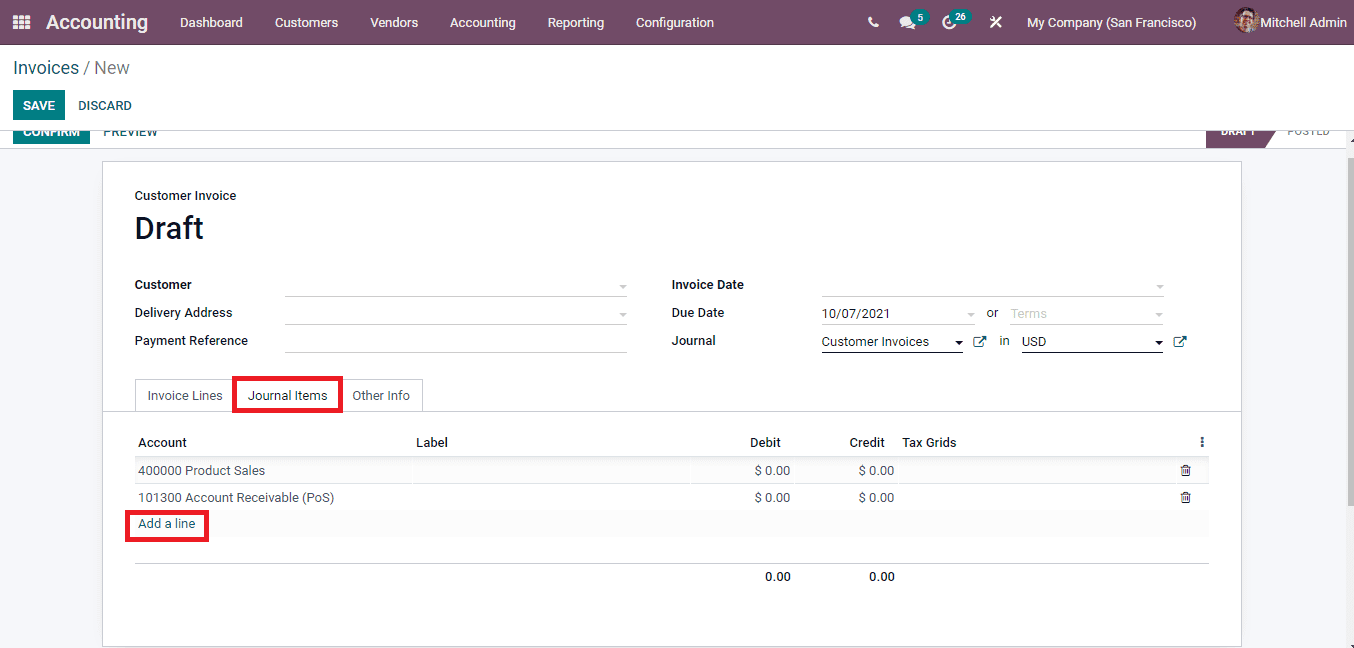**Descriptive Caption:**

This image showcases a web page interface featuring a sleek, dark purple bezel. On the left side, nine closely packed squares are prominently displayed. On the right, the word "Accounting" is rendered in bold white text, complemented by various non-bold white clickable tabs including "Dashboard," "Customers," "Vendors," "Accounting," "Reporting," and "Configuration." Adjacent to these, there are icons: a telephone symbol for calling, two thought bubbles for chat, and a teal circle with a white numeral '5' indicating five messages. Additionally, a circle with the numbers '36' or '26' (unclear) and a wrench and another tool, possibly a fork and knife, appear in white. Further along, the text "My Company (San Francisco)" is followed by a close-up profile picture of a person with black hair, light skin, glasses, and a gray suit labeled "Mitchell Admin" in white text. 

In the white section on the left, "Invoices" appears in green alongside a gray backslash and the word "New" in gray. Below, a bold teal button labeled "Save" is present next to a teal "Discard" button. Beneath these, a button reading "Confirm" is followed by a truncated "Preview" button. On the far right, a "Posted" button is followed by a purple button that is partially cut off.

Transitioning to a new white rectangle section atop a gray background, the top reads "Custom Invoice" in black, with "Draft" in bold black text nearby. "Customer" is labeled in black with an accompanying dropdown arrow, followed by "Delivery Address" and "Payment Reference" in black. To the right of "Delivery Address" is "Due Date," and next to "Payment Reference" is "Journal." Below, tabs labeled "Invoice Lines," "Journal Items" (highlighted with a red border), and "Other Info" are visible. 

In the accounting portion labeled "Account at Label," we see "400000 Product Sales" and "101300 Account Receivable (POS)" with $0 for both debit and credit values respectively. A red rectangle surrounds a "Add a line" link in blue hyperlink text. Further below, past the debit and credit sections showing $0, there are tax grids with no entries and two trash cans indicating deletable items. At the top right, an ellipsis allows for editing.

Continuing on the right, the "Invoice Date" and "Due Date" appear in bold black, with regular text indicating "10-07-2021." A dropdown arrow offering "Terms" in faded gray follows. In the "Journal" section, "Customer Invoices" is listed next to a dark blue square icon with an arrow. Finally, the text "USD" in black with a dropdown arrow appears alongside a dark blue square with an outward-pointing arrow.